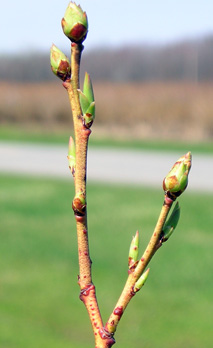This realistic, portrait-oriented photograph captures a budding plant in meticulous detail. Dominating the full height of the image, the prominently featured plant consists of two main stems: one larger stem rises almost vertically to the left, while a secondary stem branches off to the right. The plant is characterized by the absence of leaves and the presence of green, teardrop or pear-shaped buds at the stem tips. These prominent buds are encased in a darker purplish-red or dark pink casing, with hints of red and purple.

The background is a blurred, grassy, wheat field, enhancing the focus on the plant. In the middle of this blurred backdrop, a path or road is discernible, flanked by green grass that transitions to taller, darker grass or possibly a small forest in the distance. The overall composition highlights the plant's anticipation of blooming, with its intricate buds waiting to flourish against the subtly detailed, muted landscape beyond.